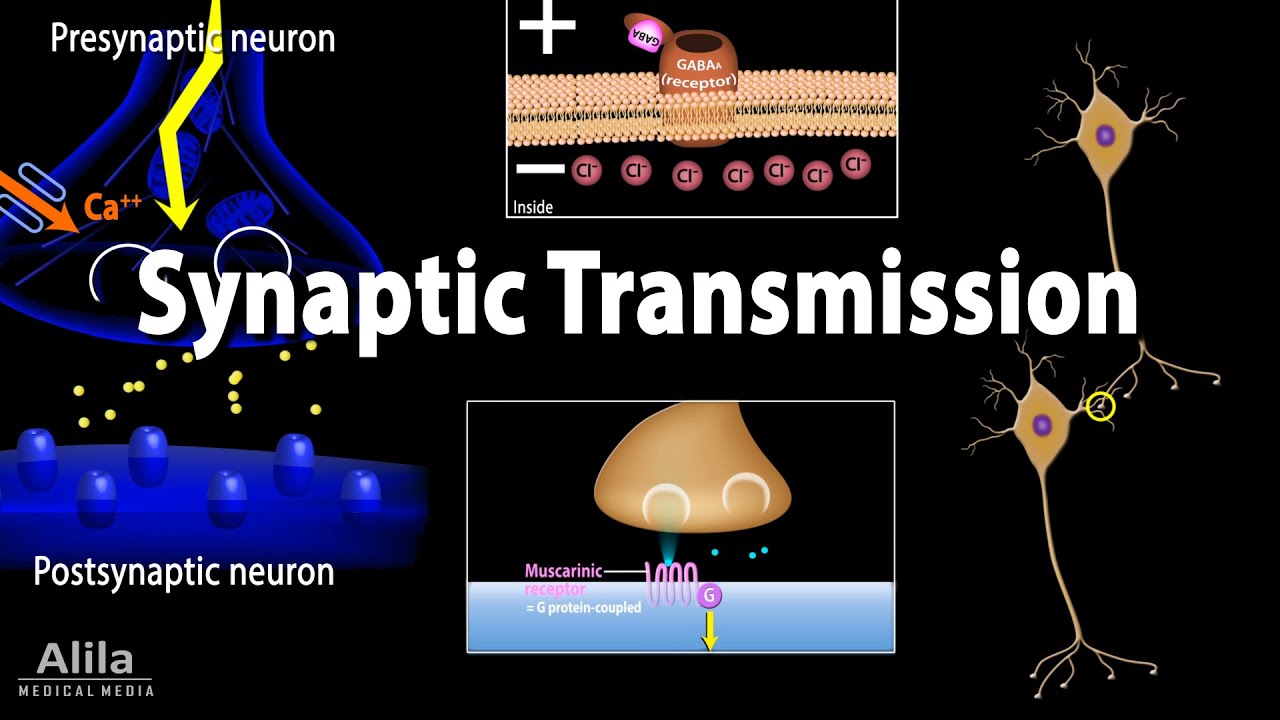This image is a detailed, digitally created diagram set against a completely black background, likely from a scientific manual, medical textbook, or a slide from a talk, presenting the process of synaptic transmission. Dominating the center in bold white text are the words "Synaptic Transmission." In the upper left, labeled "presynaptic neuron," a structure resembling a transparent blue beaker funnels yellow beaded nodules downward, illustrating neurotransmitter release. A yellow arrow labeled "synaptic transmission" points towards the "postsynaptic neuron" at the bottom right, where the neurotransmitters appear to interact with the cell's surface, depicted as blue floating buoys.

To the right, the image features two rectangular insets. The upper inset zooms into a bilipid membrane containing a GABA-A receptor, highlighting GABA alongside chloride ions indicated by plus and minus signs. The lower inset shows a muscarinic receptor, labeled "E = G protein coupled," denoting its interaction with G proteins. Brown dendritic structures and neurons frame the colorfully illustrated elements, making the diagram visually informative.

At the bottom left, the source is credited as "Alila Medical Media." The diagram, presented in landscape format, meticulously breaks down the complex biological process of synaptic transmission using both textual labels and vivid graphical depiction.